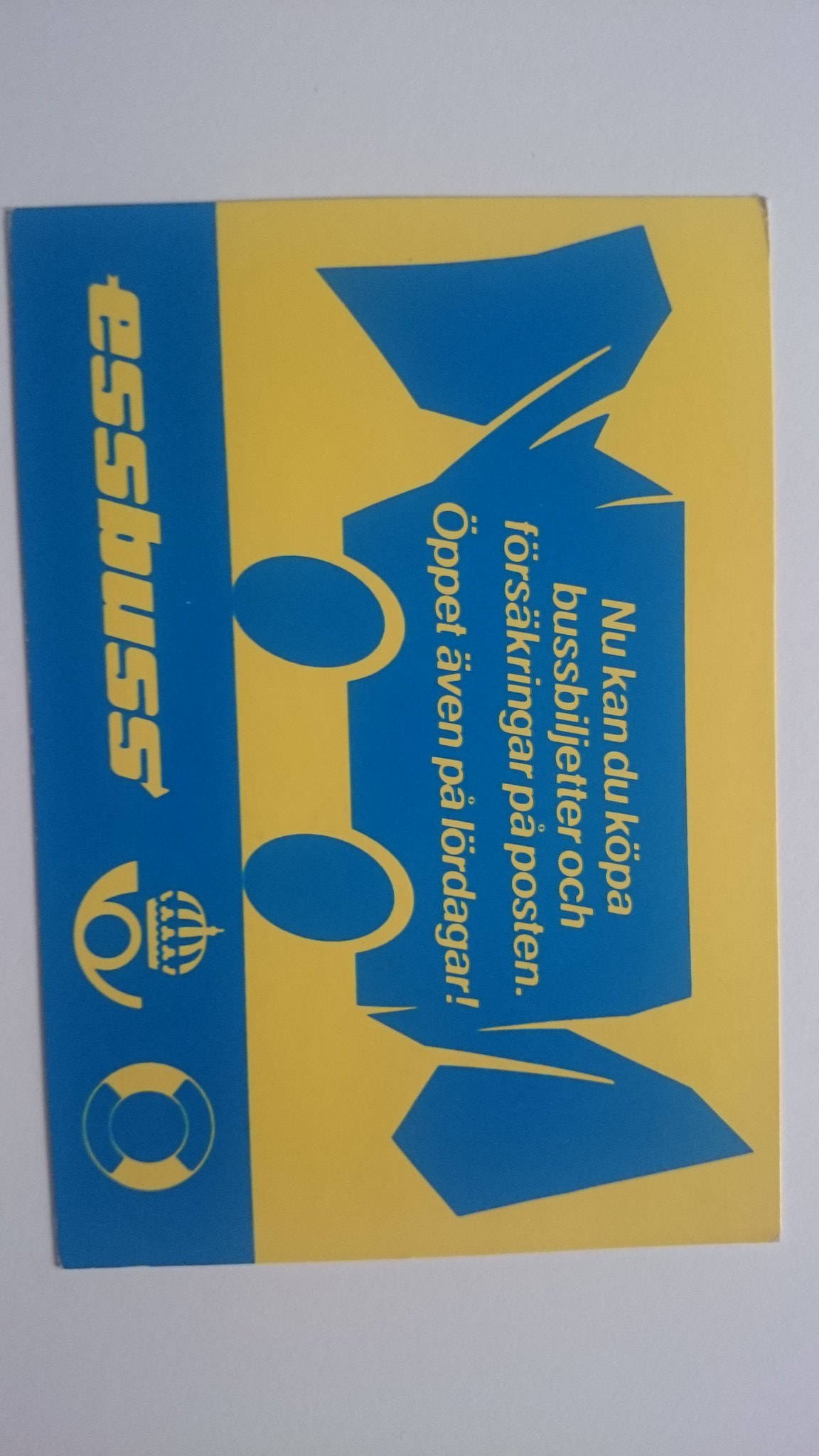This image depicts a landscape-oriented card or sign that has been photographed in portrait orientation, turned 90 degrees to the right. The card features a yellow background covering approximately three-quarters of the top section, while the bottom quarter is a bright royal blue stripe. On the yellow background, there is a simple, block-style outline drawing of a vehicle, which appears to be a tractor, digger, garbage truck, or bus, in blue. The vehicle has two blue circles underneath it, representing wheels.

Beneath this image, on the blue stripe, there is yellow lettering that spells out "E-S-S-B-U-S-S," suggesting it pertains to a bus company. Adjacent to the text are logos, featuring symbols such as a crown atop a circular object that resembles a pot. Text in a foreign language, possibly Swedish, is also present on the card, including phrases such as "Nu kan du köpa bussbiljetter och försäkringar på posten." This detailed and eye-catching design hints at a promotional or informational piece related to transportation services.